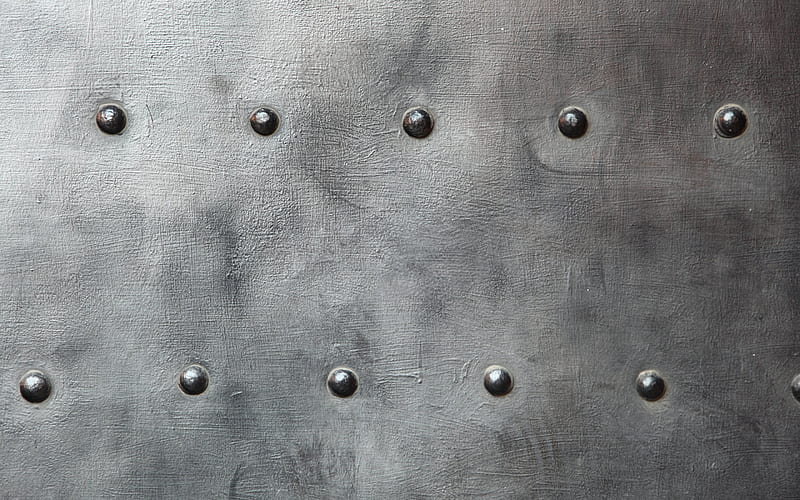This close-up photograph features a dark gray, textured material resembling leather or vinyl. The texture is interspersed with lighter and darker shades of gray, giving it a dynamic, oil-painting-like appearance. Prominently displayed are two staggered rows of rivet-like circles or silver-colored studs. Each row consists of five equally spaced studs: the top row situated about an inch from the top edge of the photo, and the bottom row about an inch from the bottom edge. The studs stand out with a dimensional quality, contributing to the overall tactile and visual complexity of the image.